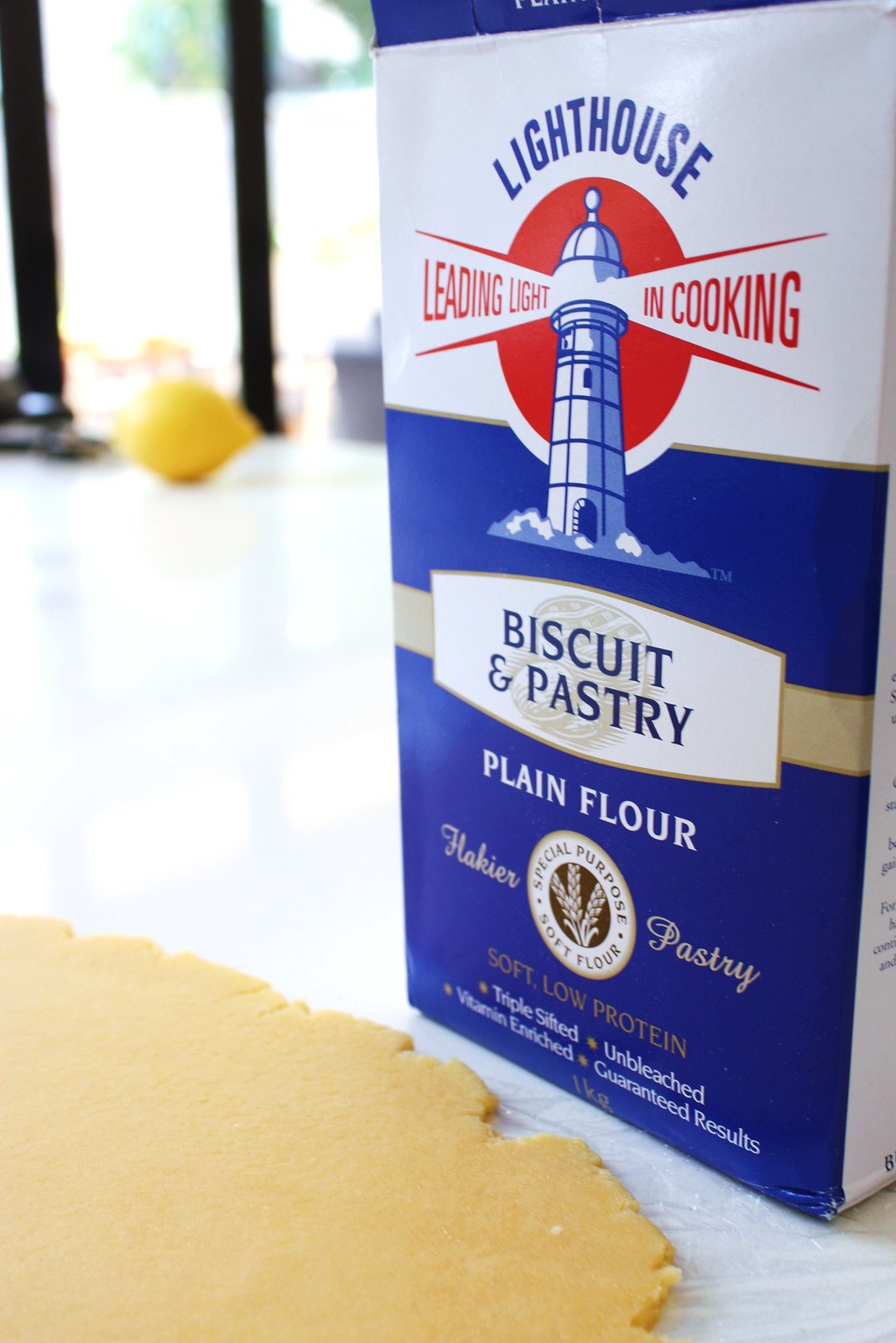This vibrant color photograph captures a close-up scene centered on a blue and white package of Lighthouse Biscuit and Pastry Plain Flour, prominently placed on a tabletop. The flour box, adorned with a lighthouse emblem and branded as the "Leading Light in Cooking," emphasizes its special-purpose, soft, low-protein quality ideal for biscuits and pastries. To the right of the box, some rolled-out pastry dough is visible, hinting at an ongoing baking endeavor. The soft background features an out-of-focus lemon, subtly adding a touch of yellow to the scene and contributing to the kitchen's warm and inviting atmosphere.